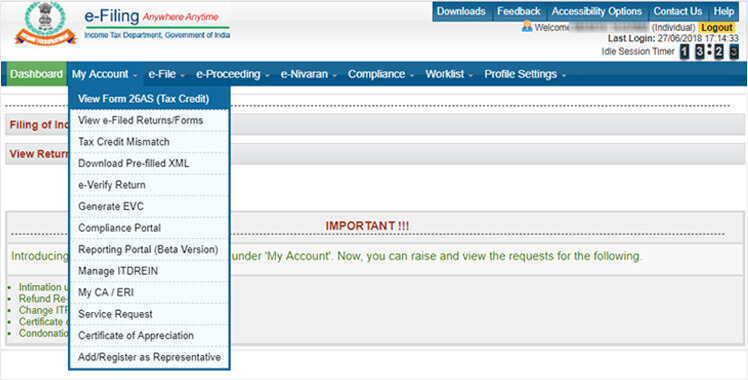This image depicts a web page interface for e-filing taxes on the Income Tax Department, Government of India’s website. 

In the upper left-hand corner, there is an emblem featuring a gray design encircled by a turquoise ring; the emblem is small and slightly blurry, making its details difficult to discern. Below the emblem, a red half-circle banner displays white text. To the right, the term "e-filing" is prominently shown with "e-" in lowercase and "FILING" in uppercase letters. Adjacent to it, in small red italicized text, is the phrase "anywhere, anytime." A green line runs beneath these elements, followed by tiny bright blue text stating "Income Tax Department, Government of India."

To the right, several tabs in dark blue with white text provide navigation options. These tabs include: Downloads, Feedback, Accessibility Options, Contact Us, and Help. Below this navigation bar, a gray text message welcomes the user, whose name is blurred out. A yellow “Log Out” button with black text stands out prominently, and information about the user's last login, dated 27-6-2018, and the corresponding time, is displayed. An idle session timer currently reads 13:23.

Below this, a bright blue banner spans the width of the page, featuring various navigation options in white text: Dashboard, My Account, e-File, e-Proceeding, e-Navarin, Compliance, Work List, and Profile Settings. The "Dashboard" option is highlighted in green with white text, and the "My Account" tab is selected, showcasing a dropdown menu with a vertical list of options such as: View Form 26AS (Tax Credit), View e-Filed Returns/Forms, Tax Credit Mismatch, Download pre-filled XML, e-Verify Return, and more.

This detailed structure indicates a well-organized and comprehensive portal aimed at facilitating seamless tax filing for users.